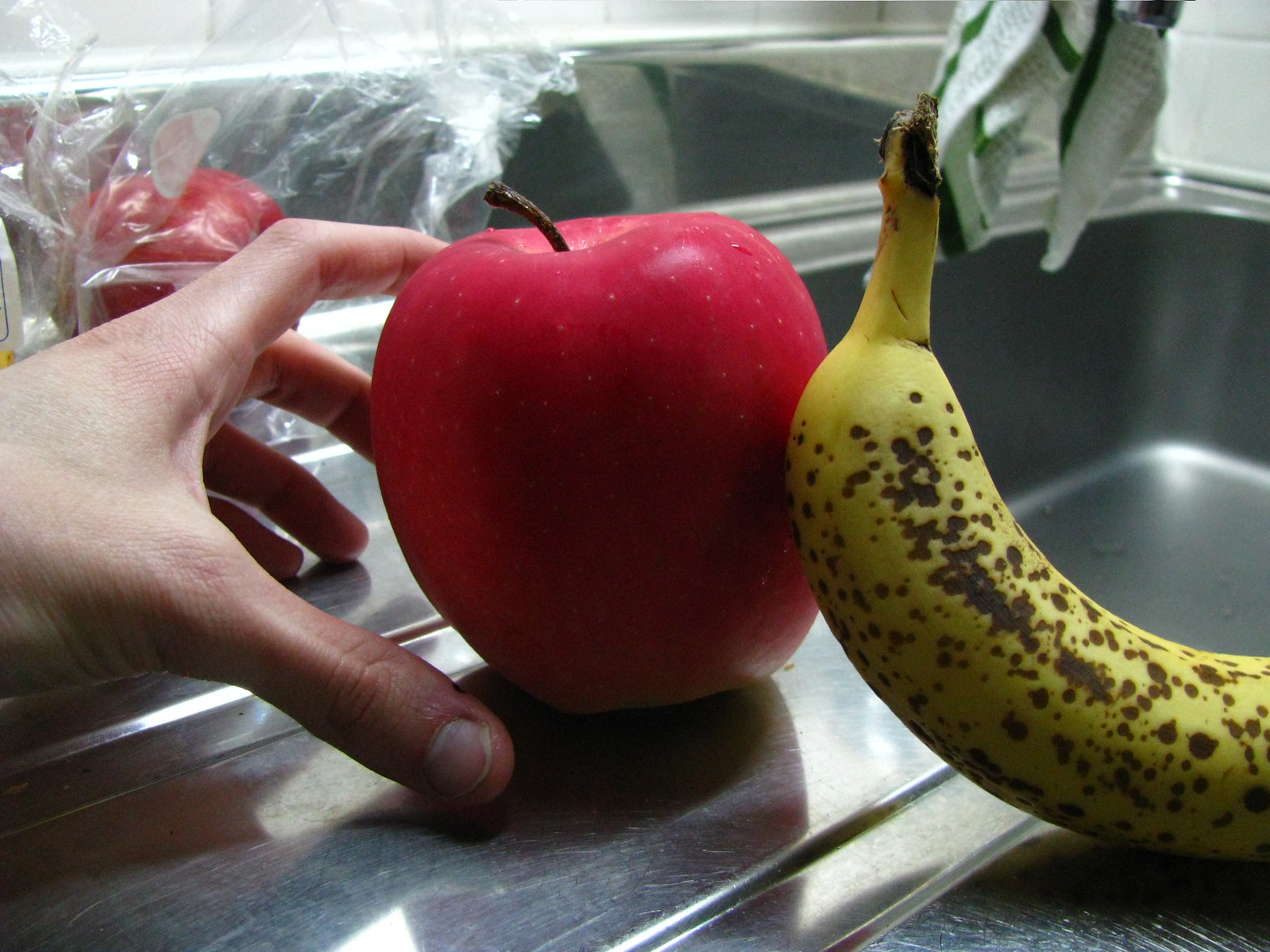In this wide-angle photograph of a kitchen setup, the focal point is a person's hand near the left center of the image holding a vibrant, cartoonishly-colored red apple. The hand, with its elongated thumb pointing downward and the index finger curved to form a 'C' shape around the apple, delicately cradles the fruit without the thumb and index finger touching. To the right of the apple, a banana with mottled brown spots rests on the metallic surface of the sink area.

The setting is a metal sink, which occupies the right side of the frame, with a raised platform on the left. A green and white dish towel is draped over what appears to be the faucet. In the upper left-hand corner of the image, a piece of saran wrap is visible, adding a subtle layer of daily kitchen activity. White, subway-style tiles adorn the very top and upper right-hand side of the photograph, adding a clean, orderly backdrop.

Apart from the hand, apple, banana, dish towel, and saran wrap, the scene is minimalistic—no dishes clutter the sink, and no other objects are visible. There is no indication of the person’s identity or gender, and their activities remain a mystery beyond this singular moment captured in the photograph.